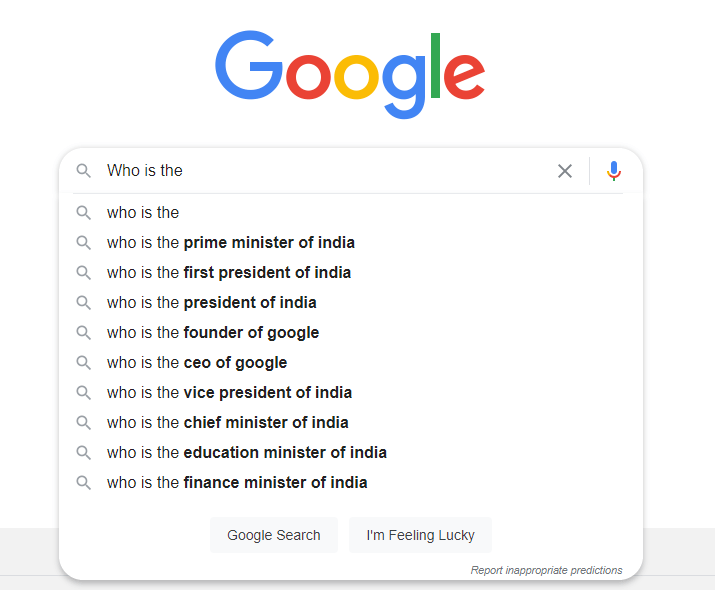The image displays a classic Google search page, characterized by its minimalist design and iconic color scheme. Dominating the top center of the white background is the "Google" logo, notably rendered in vivid hues of blue, red, yellow, and green. Below the logo, a search bar is centered, featuring pre-typed text that reads "who is the." 

This query triggers a drop-down menu of predictive search suggestions, all beginning with "who is the" in gray text followed by specific queries in black. The suggestions include:
1. Prime Minister of India
2. First President of India
3. President of India
4. Founder of Google
5. CEO of Google
6. Vice President of India
7. Chief Minister of India
8. Education Minister of India
9. Finance Minister of India

Beneath the search bar and its suggestions are two clickable buttons labeled "Google Search" and "I'm Feeling Lucky." Further down, on the right side, is a discreet link labeled "report inappropriate predictions." In the upper-right corner of the page is a microphone icon distinguished by Google's signature colors, indicating voice search functionality.

The entire interface is set against a stark, clean white background. There is a subtle gray strip at the very bottom of the page, lightly visible and marked by a thin gray line. This element enhances the visual separation without adding any content. The color palette prominently features blue, red, yellow, green, gray, white, and black, adhering to Google's branding and ensuring a clear, uncluttered user experience.